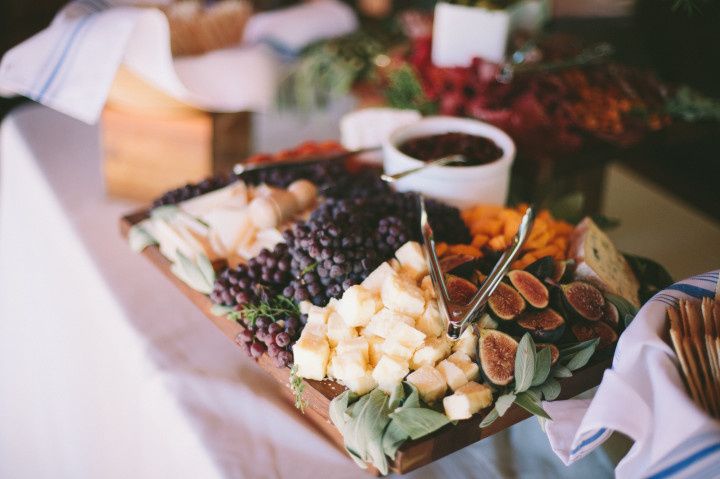The image features an angled shot of a meticulously arranged charcuterie board placed at the center of a white tablecloth-covered table. At the heart of the board are an assortment of cheeses, including white cheese, and various fruits such as halved figs displaying their red centers and purple skins, along with clusters of grapes. The board is accentuated with sprigs of green rosemary, adding a touch of freshness.

Accompanying the main components, a pair of shiny metallic tongs rests atop the assortment, facilitating easy serving. Nestled among the offerings is a white ceramic bowl containing a dark reddish sauce or marmalade, complete with a silver spoon for serving. To the right, there’s a bowl that is partially visible, covered with a white napkin adorned with blue stripes, hinting at crackers inside.

Blurry elements populate the background, hinting at additional servings and a lively setting, possibly indicating a fancy gathering or party such as a wedding. The table also features more white napkins with blue stripes, adding a consistent design element. Though some details remain indistinct due to blurring, the overall composition evokes a sense of elegance and attention to detail.